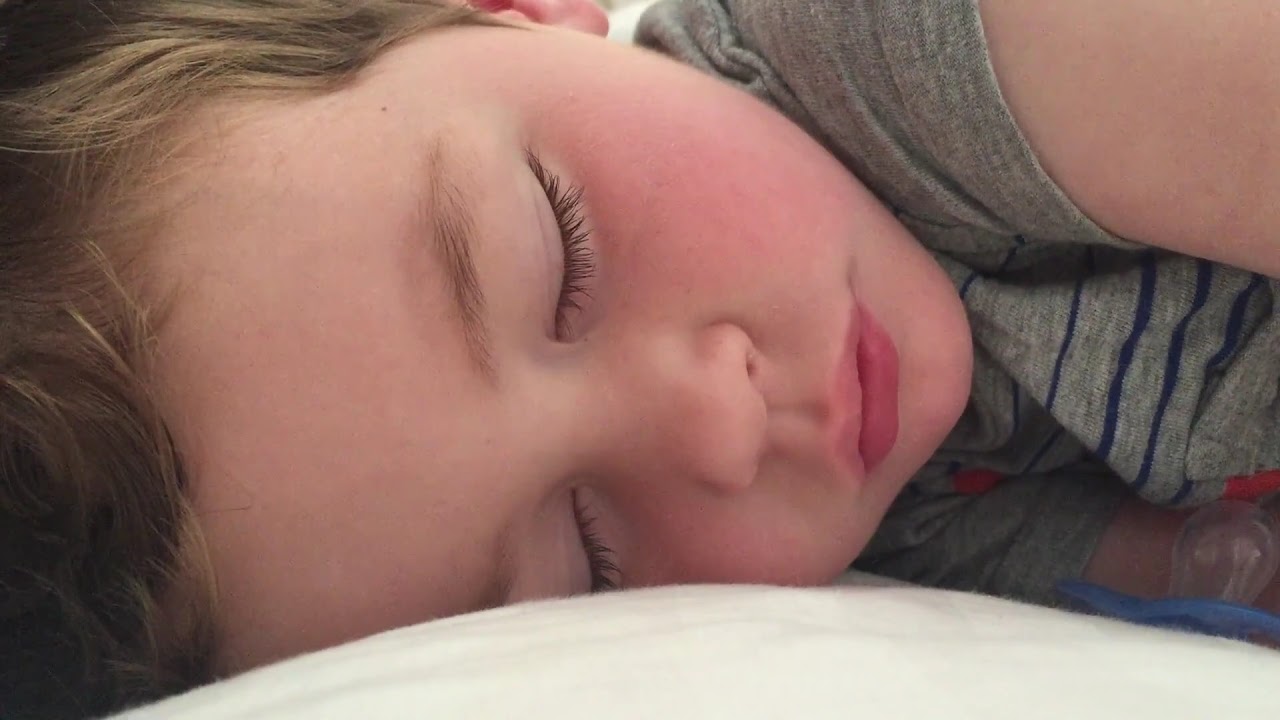This image captures a close-up of a peacefully sleeping Caucasian toddler boy, approximately two to three years old. The main focus is on his cherubic face with eyes closed, framed by slightly wavy sandy blonde to light brown hair, and adorned with brown eyebrows and long dark lashes. His pink rosy cheeks and rosebud lips add a tender touch to his serene expression. His head rests on a soft white or cream-colored pillow or sheet, occupying most of the picture, while his body is oriented sideways with his head to the left of the frame. He is clad in a gray t-shirt with thin blue stripes that resemble painted strokes, typical of contemporary style. A blue pacifier with a white nip can be seen near his right arm. The scene is brightly lit, suggesting it was taken during the daytime, capturing the innocence and tranquility of the sleeping child.